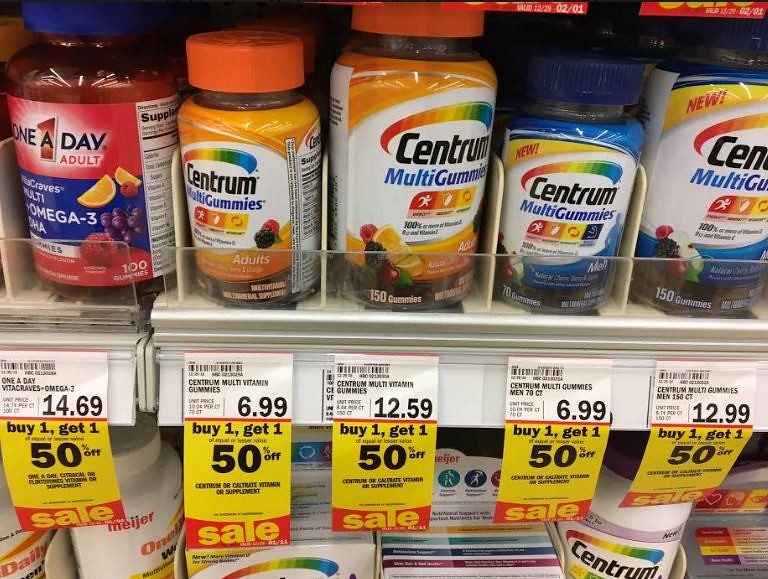The image captures an aisle inside a store filled with a variety of multivitamin bottles and boxes neatly arranged on shelves. On the top shelf, there are five distinct sections. The first section features a "One A Day Adult" multivitamin in a red bottle. The second section showcases an orange bottle of "Centrum Multigummies". The third section contains a larger orange bottle of "Centrum Multigummies". The fourth section displays a blue bottle of "Centrum Multigummies", followed by a larger blue bottle in the fifth section.

Each bottle has a corresponding price tag beneath it. The original prices are printed in white, and there's a prominent promotional offer highlighted in yellow and red: "Buy One, Get One 50% Off". 

Below the top shelf, the bottom shelves are filled with a mix of bottled and boxed vitamins. The first two items are regular white bottles. The subsequent sections alternate between boxed and bottled vitamins, making a total of six rows at the bottom. The boxes are predominantly white, adorned with multicolored designs and images of fruits and vegetables, emphasizing health benefits. To the right of the white bottles, there's a white Centrum bottle followed by another box, maintaining the vibrant and colorful theme present throughout the display.